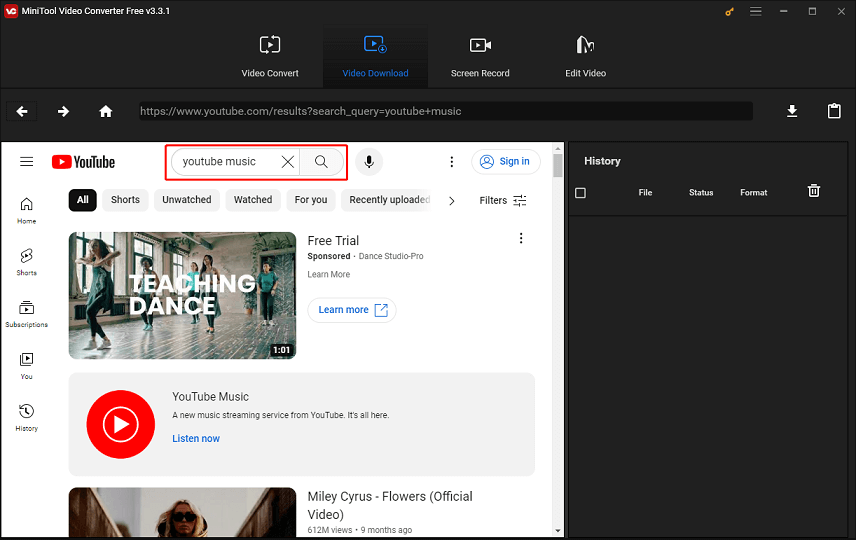This is a detailed screenshot of the MiniTool Video Converter Free version 3.3.1 application. The application interface features a dark gray background and prominently displays a web page in the bottom left section of the frame.

In the top left corner, there is a header with a red square icon with rounded corners marked "VC" in white. To the right of this icon, the application title "MiniTool Video Converter Free v3.3.1" is displayed. In the top right corner of the header, there is a series of icons: a gold key icon, followed by three light gray icons depicting three horizontal lines stacked vertically (menu), a minus icon (minimize), a square icon (maximize/restore), and an X icon (close).

Beneath this header, centrally located in the frame, are four main tabs for navigating through the application. From left to right, the first tab features two white arrows in a circular motion with a white triangle pointing to the right, labeled "Video Convert." The second tab, which is selected, exhibits a blue triangle with a blue outline, featuring a blue plus sign in the bottom right corner and is labeled "Video Download." The selected state is indicated by a gradient gray box that is darker at the bottom and lighter at the top. The third tab showcases a cinema camera icon with a white triangle, labeled "Screen Record." The fourth tab features a 3D-style "M" outline in white, labeled "Edit Video."

Directly below these tabs is a thin black line that separates them from the URL bar below it. The URL bar is centered within a black header, containing the white text "https://www.youtube.com/results?search_query=youtube_music." Additional icons are present to the right of this URL bar but are not described in detail.

The highlighted web page displayed in the bottom left corner of the frame is a YouTube page with a white background, effectively integrating into the application's interface for web-based video searches and downloads.